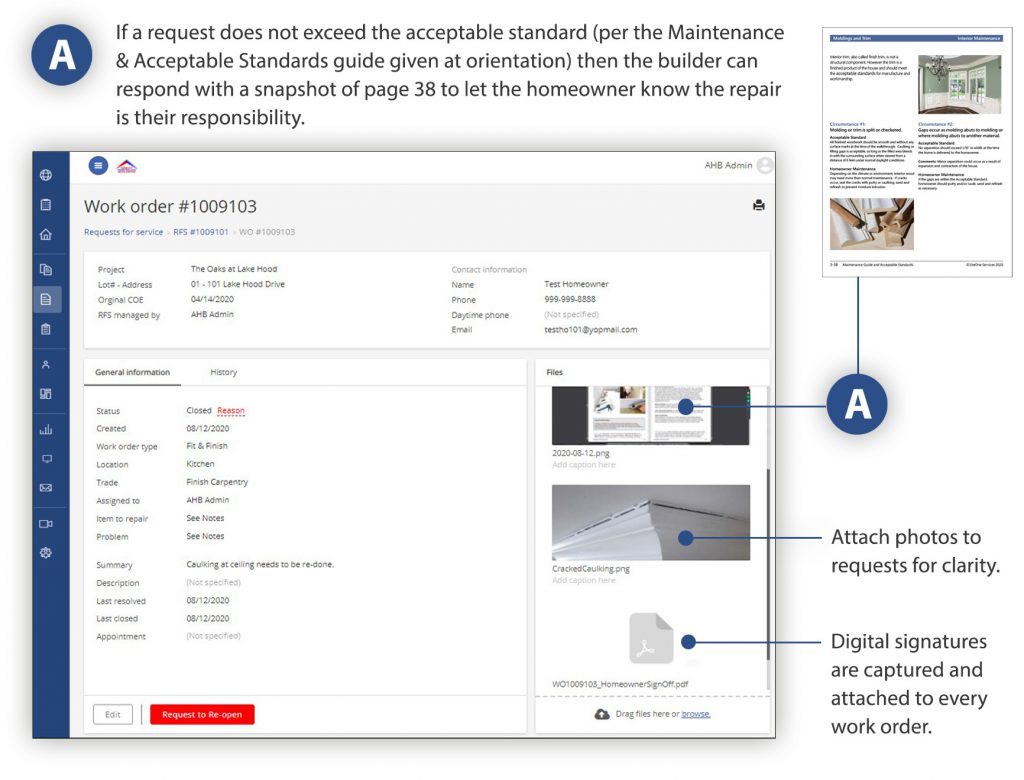This digital image is a detailed screenshot of a desktop computer program, displayed against a white background. The main focus, occupying approximately three-quarters of the screen in the bottom left corner, is a web page interface.

In the top left corner, an eye-catching blue circle with a white capital "A" sits prominently, casting a medium gray shadow behind it. Adjacent to this blue circle is a paragraph of carefully structured black text, extending across the remaining width of the web page. The text meticulously explains: "If a request does not exceed the acceptable standard (per the Maintenance and Acceptable Standards Guide given at orientation), the builder can respond with a snapshot of page 38 to inform the homeowner that the repair is their responsibility."

To the right of this primary web page, another screenshot of a separate website is visible. This secondary screenshot features a clean white background and a blue header, accompanied by a couple of interior photos and several lines of black text, presenting additional context or information.

Below this second screenshot, a dark blue line runs horizontally from its bottom left side, connecting to another blue circle featuring a white "A" and casting a similar shadow. A horizontal dark blue line extends leftward from this second circle, leading back to the initial web page, terminating in a small dark blue circle.

Below the second blue circle, two succinct lines of black text instruct: "Attach photos to requests for clarity." Continuing the visual journey, another blue line and circle arrangement extends leftward, with four more lines of informative black text below: "Digital signatures are captured and attached to every work order." This section also features a parallel blue line and circle configuration, running back towards the web page, seamlessly integrating all elements of the visual guide.

The intricate labyrinth of lines, text, circles, and screenshots effectively communicates the process flow within the program, providing a comprehensive visual representation of how information is interconnected and conveyed.